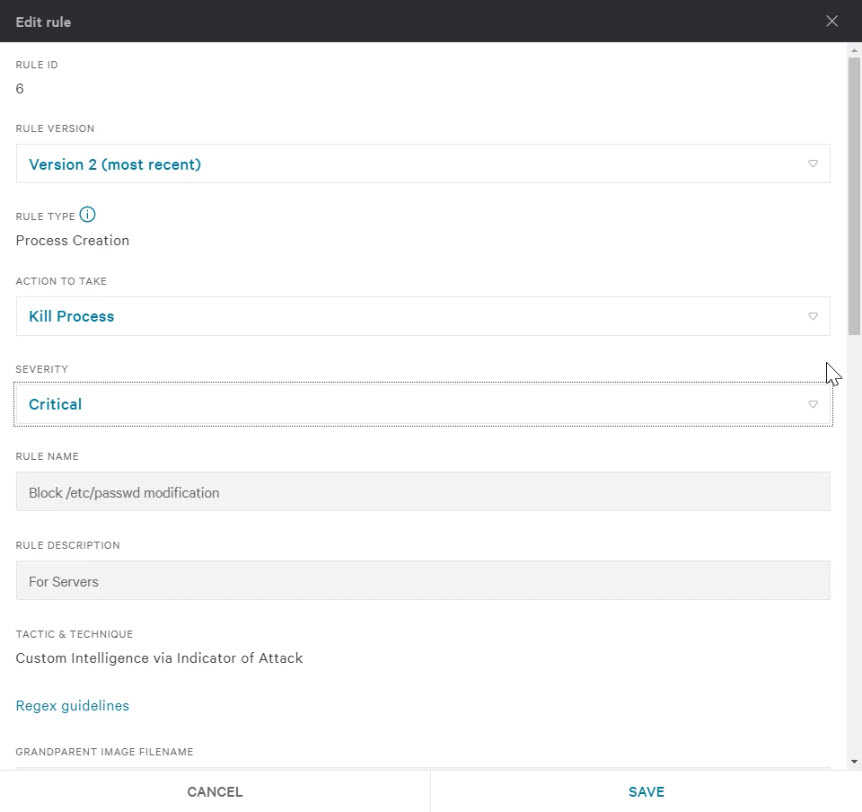**Caption:**

A detailed screenshot of a computer program interface titled "Edit Rule." The top section features a black horizontal banner with "Edit Rule" in white text on the left and a white "X" on the right. Along the right edge, a light and dark gray scroll bar signifies the presence of more content below the visible area. 

The interface begins with the label "Rule ID" followed by the number six. Below that, “Rule Version” is displayed alongside a drop-down menu indicating "Version 2" with "most recent" in parentheses, highlighted in a bluish-teal color. 

Next is the "Rule Type" field, which has an information icon in blue next to it, displaying "Process Creation." This is followed by "Action to Take," where a drop-down search box shows the text "Kill Process" in blue. 

Following this, there is a "Severity" section with a dropdown indicating "Critical" in blue text. The "Rule Name" field contains the text "Block /etc/passwd modification." The "Rule Description" field shows "For Servers." 

Subsequently, "Tactic and Technique" is labeled with the description "Custom Intelligence via Indicator of Attack." There is also a blue link labeled "Rejects Guidelines.” 

The final part of the interface features a label “Grandparent Image File Name” accompanied by fields that can be altered. At the bottom of the interface, there are two buttons: "Cancel" and "Save."